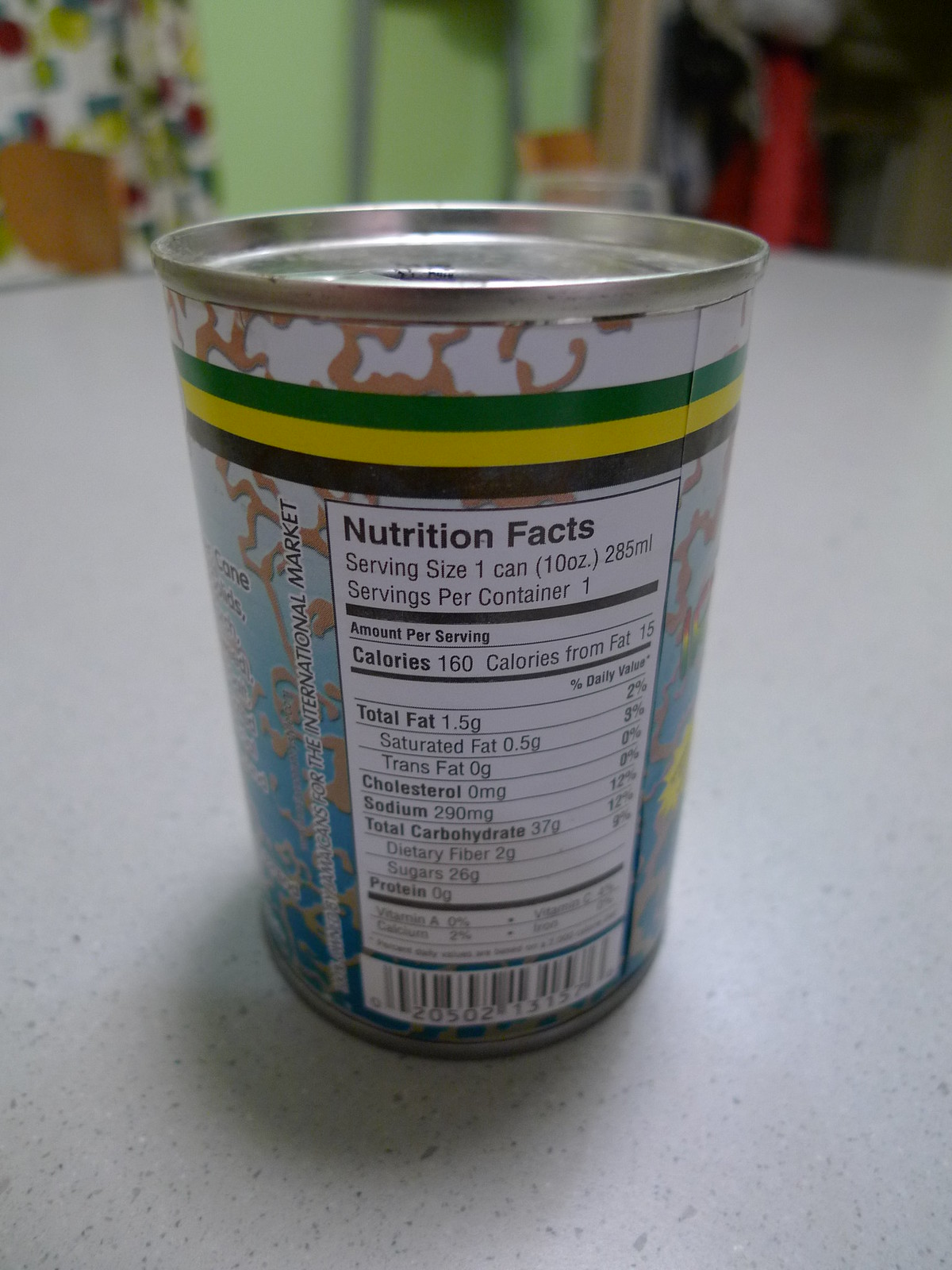The image depicts a traditional aluminum can of food, resting on a light gray countertop with tiny blue-gray spots. The can features a silver top and bottom and is wrapped in a label that transitions from white at the top to blue at the bottom. Adorning the label are swirling brown patterns mixed with stripes of green, yellow, and brown bands. 

The focal point of the image is the nutritional information displayed on the back of the can. A long white rectangle prominently shows 'Nutrition Facts' in black text, revealing that the serving size is one can (10 ounces, 285 milliliters), with 160 calories per serving. Noteworthy nutritional details include 15 calories from fat, 1.5 grams of total fat, 0.5 grams of saturated fat, 200 milligrams of sodium, 37 grams of carbohydrates, with 26 grams being sugars, and 2 grams of dietary fiber, but no protein or cholesterol.

In the backdrop, a lime green wall or space provides a vivid contrast, with possibly a green door and a white curtain featuring colorful circular designs visible. Additionally, a shelf with a red towel or jacket hanging from it can be seen towards the right side of the image.